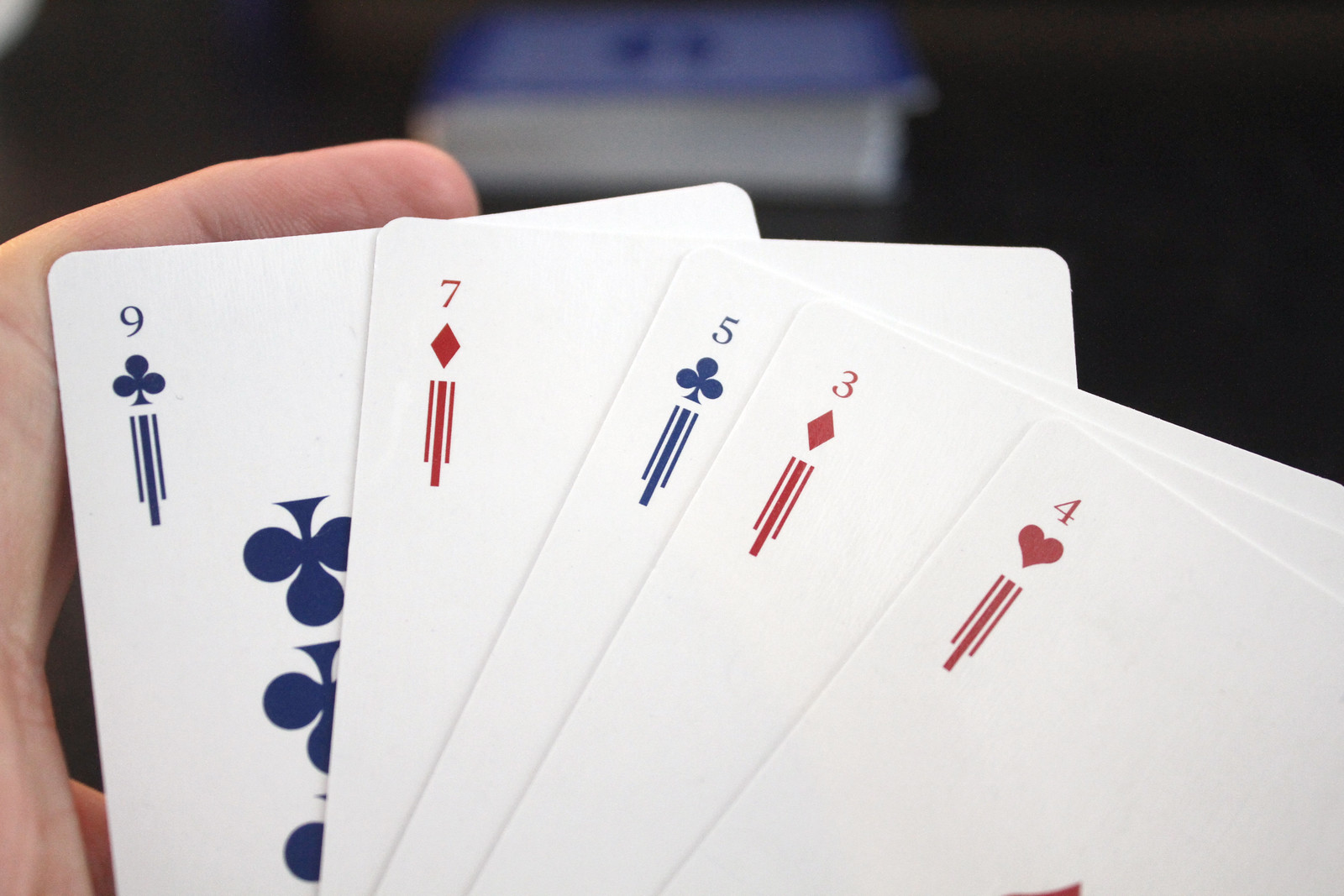This horizontally oriented rectangular image captures a segment of a person's hand on the left side of the frame. The hand is partially extended, with one finger almost parallel to the top-left edge and the rest of the hand extending vertically. The person is holding a fan of playing cards that are predominantly white and rectangular.

The foremost card displays a navy blue number '9' accompanied by a clover symbol and three vertical lines below it. The first and third lines converge at the bottom, while the middle line is thicker and extends lower. This card also illustrates three clover symbols, the first being fully visible. The second clover is partially obscured by the subsequent card, leaving only half visible, and the last clover appears as a mere dot due to another overlapping card.

The next card in the sequence is a red number '7' with a red diamond symbol beneath it, maintaining the same pattern of three vertical lines with the middle one being bolder and longer. Following this is a navy blue '5' card with a clover and the vertical lines, succeeded by a red '3' card featuring a red diamond and the vertical lines, and lastly, a '4' card showcasing a red heart and the familiar vertical line pattern.

A sliver of another red element is partially cut off at the bottom right of the '4' card, and the background of the image is entirely black, except for a distinct detail at the center of the top edge, which appears to be a combination of navy blue and white.